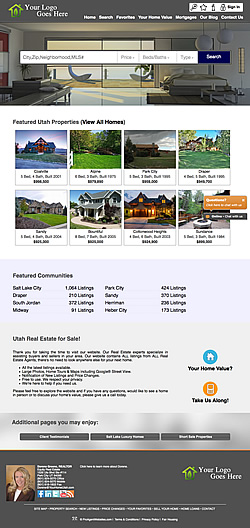This screenshot appears to be from a mobile device, displaying a prototype of a real estate website. The upper left corner is designated for the company logo, followed by navigational buttons labeled "Home," "Search," "Favorites," "Mortgage," and "Contact Us." Below the navigation bar is a search feature with fields to input city, zip code, street, price, and property type, accompanied by blue "Search" buttons. The background portrays what looks like a spacious bedroom with large deck doors opening to the outside.

Further down, there's a section titled "Featured Utah Properties" with a link to "View All Homes." This area showcases a variety of homes, including colonial and cottage styles, which are indicated to be quite expensive. Below this, there is a "Featured Communities" section listing several Utah locations: Salt Lake City, Draper, South Jordan, Midway, Park City, Sandy, and Heber City. The footer reads "Utah Real Estate for Sale," confirming the site's focus on real estate transactions within Utah.